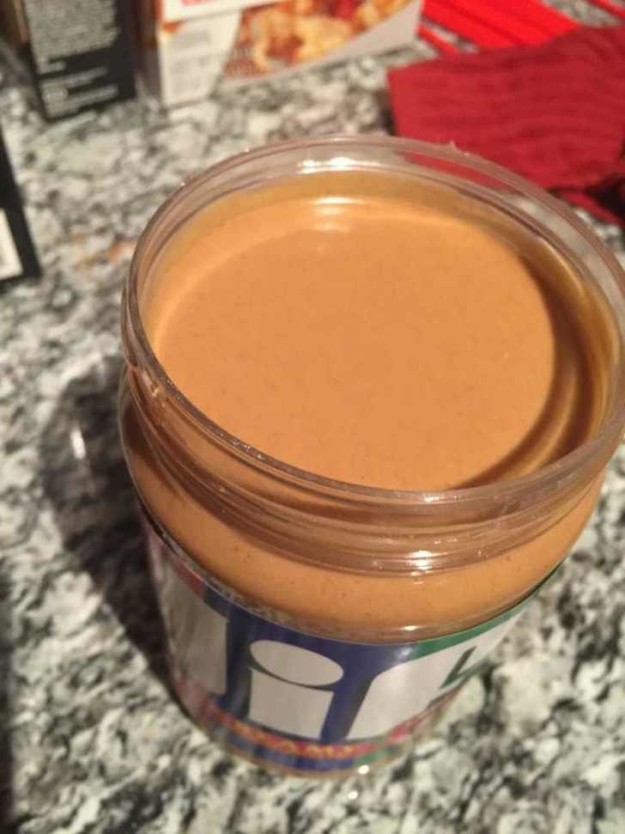The image captures a downward angle view of a freshly opened plastic jar of Jif peanut butter, sitting on a granite countertop characterized by mixed shades of gray, black, and white. The peanut butter is smooth, untouched, and a creamy orange-brown color. The Jif label prominently features vertical stripes of red, blue, and green, with the white letters "J-I-F" prominently displayed. Beside the jar, a burgundy dish towel is evident. In the background, there are various boxes, including one on the top left which is black with white, blurry text. Overlaying these boxes is another white box with brown design elements. The scene is set on a countertop that combines black parts, light, and cream-white design accents.